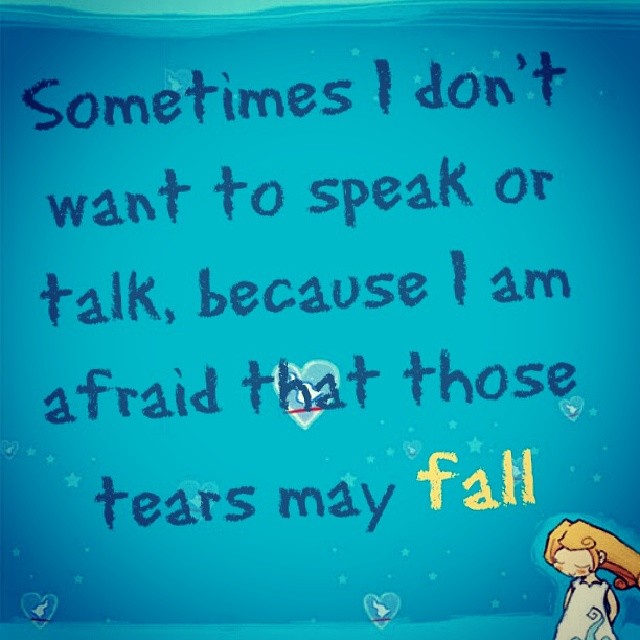The image is a square digital artwork featuring an emotional quote against a deep blue, star-studded background. Tiny light blue five-pointed stars are sprinkled across the entire canvas, while thin lines of light turquoise wave across the top, complemented by similar lines at the bottom. Several light green hearts adorned with white squiggles appear at the bottom, adding to the intricate design. Dominating the bottom right corner is a charming cartoon illustration of a young girl with white skin and curly blonde hair. She is depicted with her eyes closed, wearing a white dress adorned with blue swirls, and sporting a gentle smile with rosy cheeks. The heartfelt quote is written in a crayon-like font that mimics hand-drawn text, reading, "sometimes I don't want to speak or talk because I am afraid that those tears may fall." Notably, the word "fall" stands out in yellow, contrasting with the otherwise dark blue text. This detailed composition merges visual elements with poignant words, creating a touching piece of digital art.